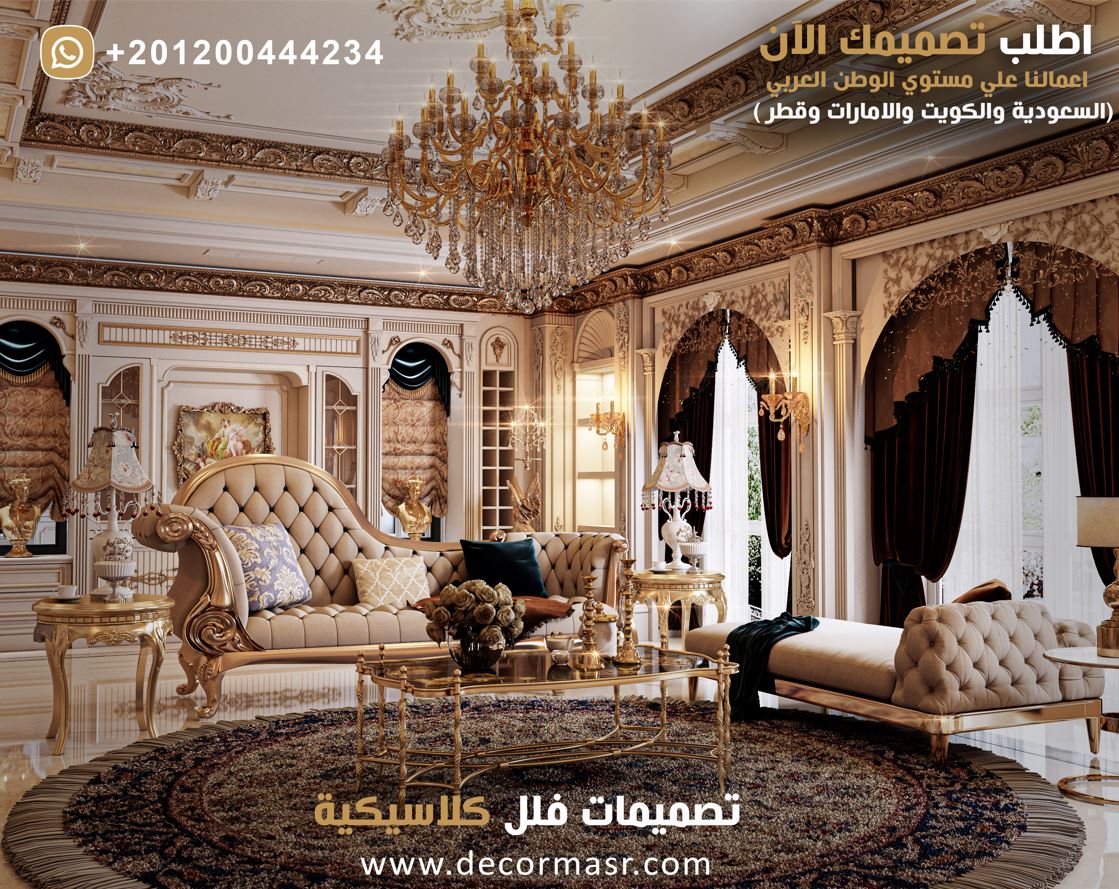This image depicts the lavish interior of a high-class living room or hotel suite, showcasing opulent Arabic decor. Dominating the scene is a grand circular rug upon which rests a glass-topped coffee table framed by two plush, tufted couches, one of which is a matching lounge. The space is adorned in a palette of cream, gold, brown, and tan. Rich velvet and brocade curtains, paired with sheer linens, dress the arched windows, which are topped with intricate gold crown molding and a golden valance. The high ceiling, painted in off-white, hosts an ornate gold chandelier dripping with crystals. Gold accents abound, including golden busts, side tables, and lamps with fringe, as well as additional golden candle holders mounted on the walls. Detailed shelving on the back wall holds various decorative elements. An Arabic text is visible in the top right corner of the image, while a phone number, +201200444234, is seen in the top left. The bottom of the image contains the URL www.decormasr.com. The overall atmosphere is one of extreme luxury and sophistication, suggesting a setting in either an upscale Arabic mansion or a deluxe hotel suite.